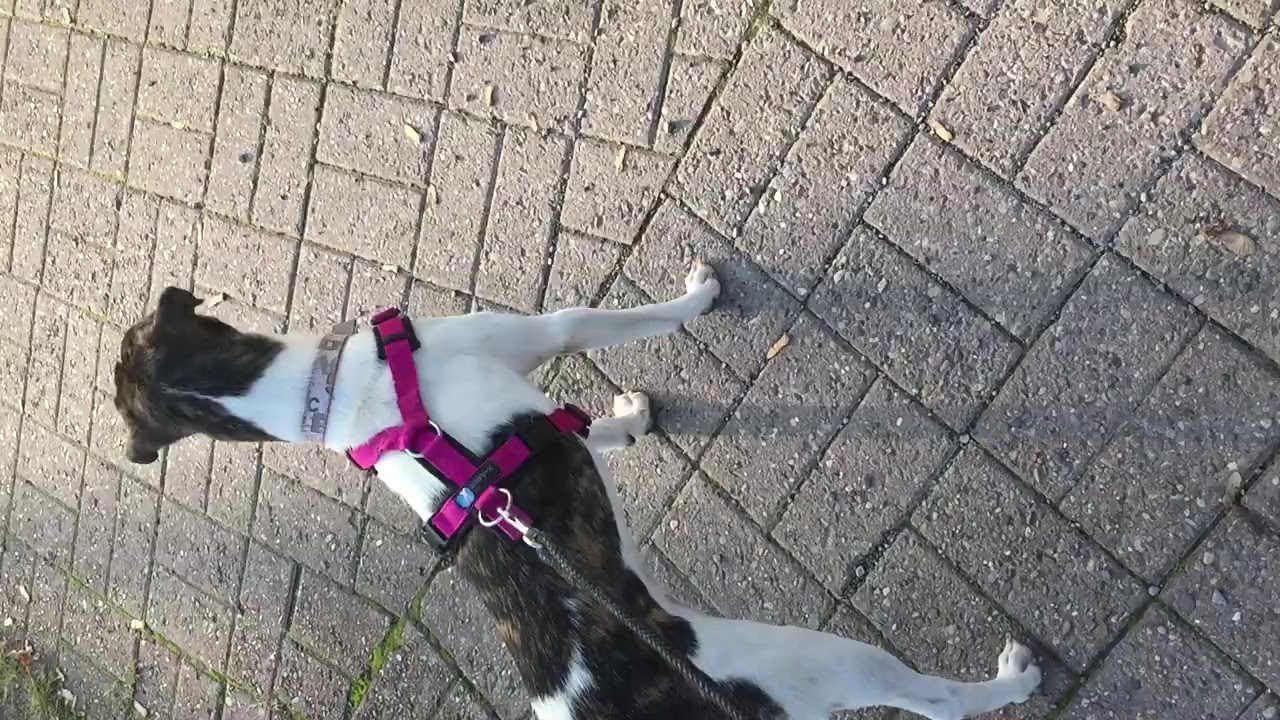In the image, we see a white dog with a distinct brindle pattern in brown hues, viewed from a diagonal top-down angle. The dog's body is oriented towards the left, with its head pointed to the left middle edge of the frame, while its body extends to the right. Its head and lower body exhibit a darker, brindle brown color, whereas its neck, front, and legs are predominantly white. The dog is wearing a bright pink or magenta harness around its shoulders and stomach, enhancing its slender frame. Attached to this harness is a black leash extending out of the frame, hinting at a connection with the person taking the photograph. Below the harness, there is a light gray strap around its upper chest just below the transition from white to dark fur.

The scene is set outdoors on a paved area with an intricate pattern of rhombus-shaped and rectangular gray tiles. Some grass sprouts through the cracks between the tiles, adding a touch of nature to the urban setting. The sunlight illuminates the scene, indicating a clear daytime capture, and the overall atmosphere is calm and serene.